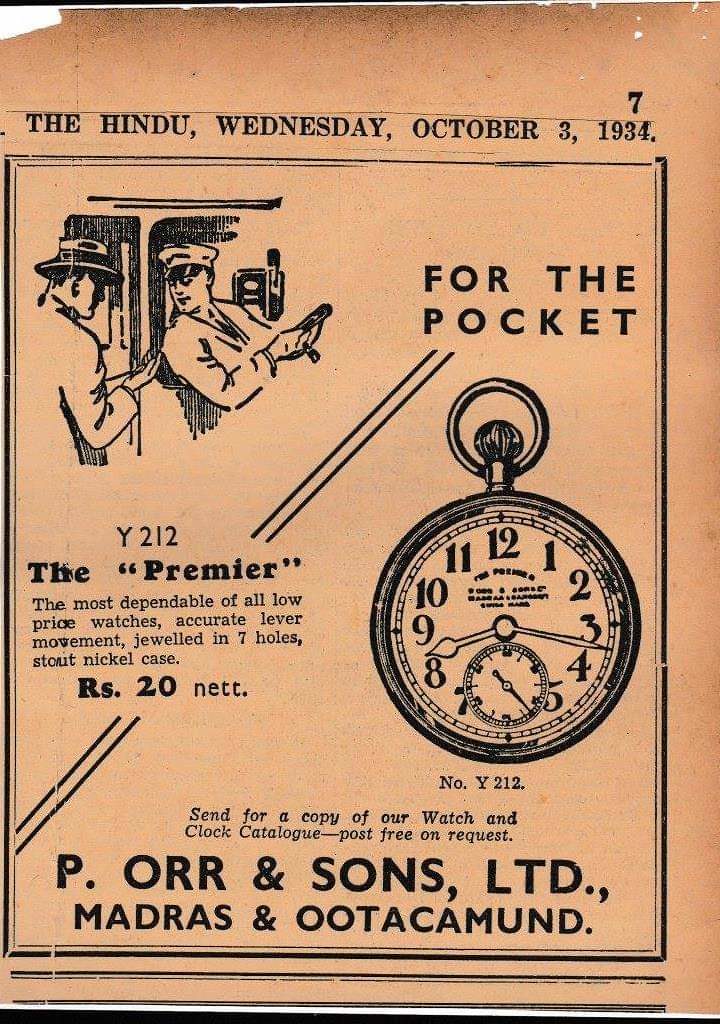The image is from an old-school advertisement, possibly from a vintage newspaper or magazine, and it has a distinct sepia tone, indicating its age. The paper is beige in color. At the very top, it reads in black letters, "The Hindu, Wednesday, October 3rd, 1934," with the page number "7" prominently displayed in the upper right corner. Enclosed within a black-bordered frame, the advertisement features an image in the upper left corner of a bus or trolley driver in uniform, with another man standing behind him, possibly showing something in his hand. Behind them, a door and some controls are visible.

Adjacent to this image, the text "For the Pocket" is clearly written. Below this text, there's a detailed illustration of a pocket watch. The watch is circular with a top ring and displays all twelve numbers along with a minute and hour hand, and a smaller dial inside with a single stick and numbers. 

To the left of the watch, detailed text describes the product: "Y212, the premier, the most dependable of all low-priced watches, accurate lever movement, jeweled in seven holes, stout nickel case, RS-20 net." Below this description, further text offers additional details, including an invitation to "send for a copy of our watch and clock catalog post free on request." The advertisement concludes with the name "P. Orr & Sons Ltd., Madras and Uttakammand" at the bottom.

This detailed advertisement showcases a reliable, cost-effective pocket watch available in 1934, presented in a periodical with clear, black text and graphics.